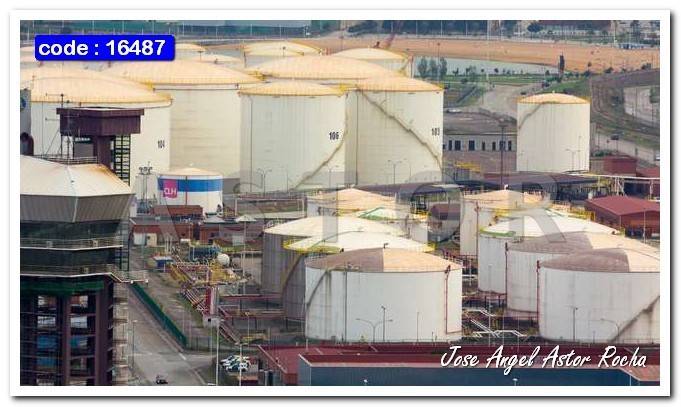This image appears to be an aerial color photograph of an industrial area resembling a postcard. In the bottom right-hand corner, the names "Jose, Angel, Aster, Roca" are written in white lettering. The upper left-hand corner features a blue rectangle with the text "code: 16487" in white letters. The foreground is dominated by numerous white cylindrical structures, some with light yellow domed tops, resembling silos used for storing corn. 

In the background, there are visible roads, a small body of water, several trees, and some cars scattered throughout the scene. Additionally, there's a red building and a larger brown building to the left, which has numerous windows, multiple stories, and an exterior staircase. A cleared field is noticeable in the upper right-hand corner. There's also a small watermark reading "A-S-T-O-R" overlaying the image. The overall scene is devoid of any people and includes a few grassy areas.